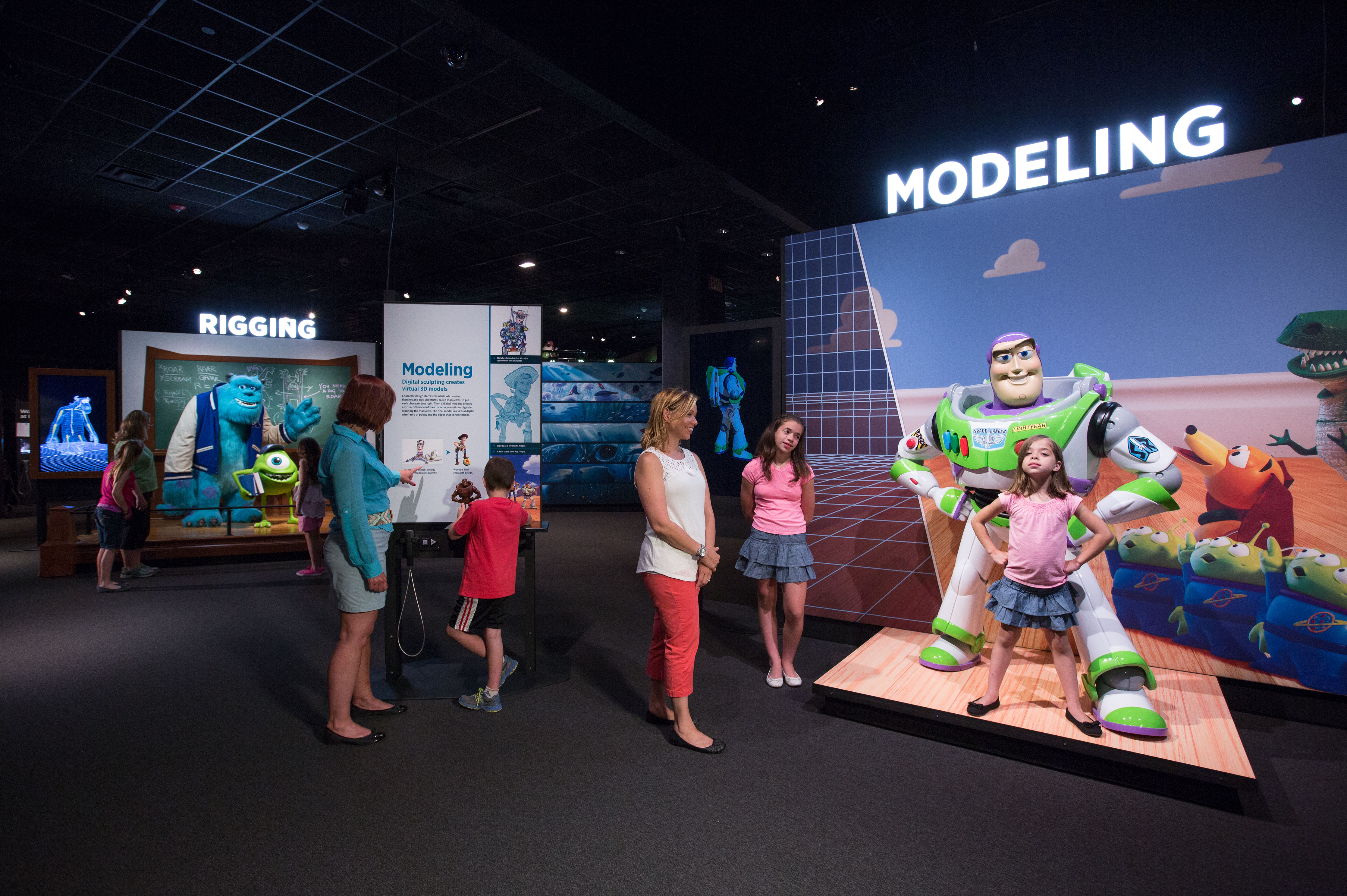This captivating photograph showcases a bustling exhibit at what appears to be Pixar Studios, where families with children are exploring various displays dedicated to Disney Pixar characters. Central to the scene is an engaging exhibit titled "Modeling," featuring a life-sized statue of Buzz Lightyear from Toy Story. One young girl stands confidently in front of Buzz, mimicking his iconic hands-on-hips pose while beaming at the camera. Her spontaneous imitation brings smiles to the faces of nearby parents and children, including her own mother and sister, who watch proudly. 

In the background, another prominent exhibit displays characters from Monsters Inc., with educational signs explaining the rigging process in animation, showing the blue ape-like Sulley and the one-eyed green Mike Wazowski in a classroom setting. Additional informational posters and demonstration boards spread throughout the spacious, high-ceilinged venue, detailing the complex processes behind character creation. This immersive environment, filled with detailed diagrams, textual information, and audio description booths, offers an enriching experience for the visiting families, highlighting the beloved Pixar characters and the artistry involved in bringing them to life.